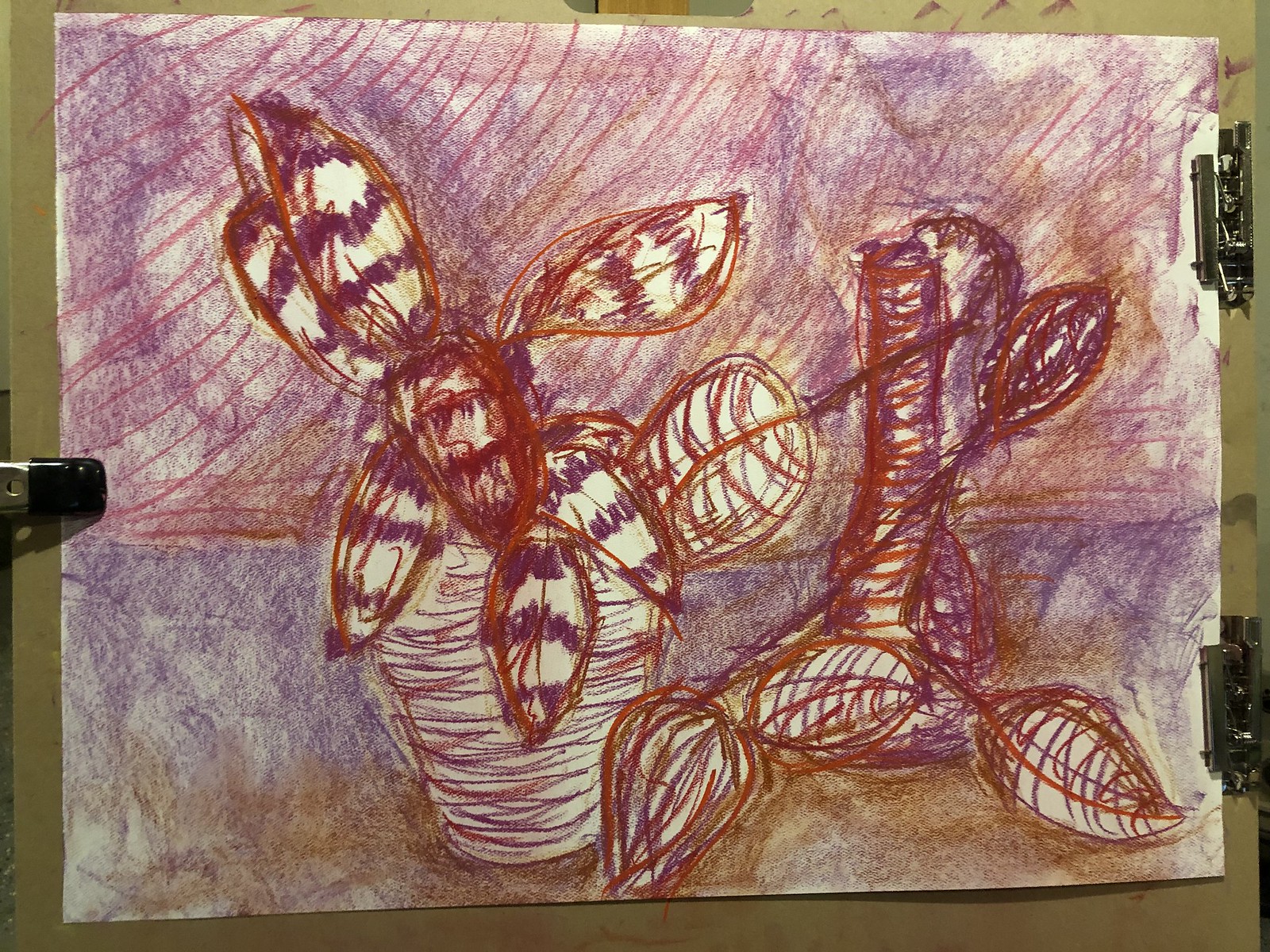The image showcases an intricately detailed drawing secured on a green drawing board, clipped on three sides for stability. The artwork itself features two hand-drawn vases, each containing a distinct plant. The first vase holds a plant adorned with lush, vibrant green leaves that appear robust and well-maintained. In contrast, the second vase contains a plant with smaller leaves that have succumbed to gravity, cascading down and resting on the ground. The background of the drawing is meticulously crafted, depicting a clear horizon and descending lines that suggest a sky, adding depth and context to the scene. The combination of thriving and wilting plants along with the nuanced background, highlights a captivating narrative within this artistic composition.